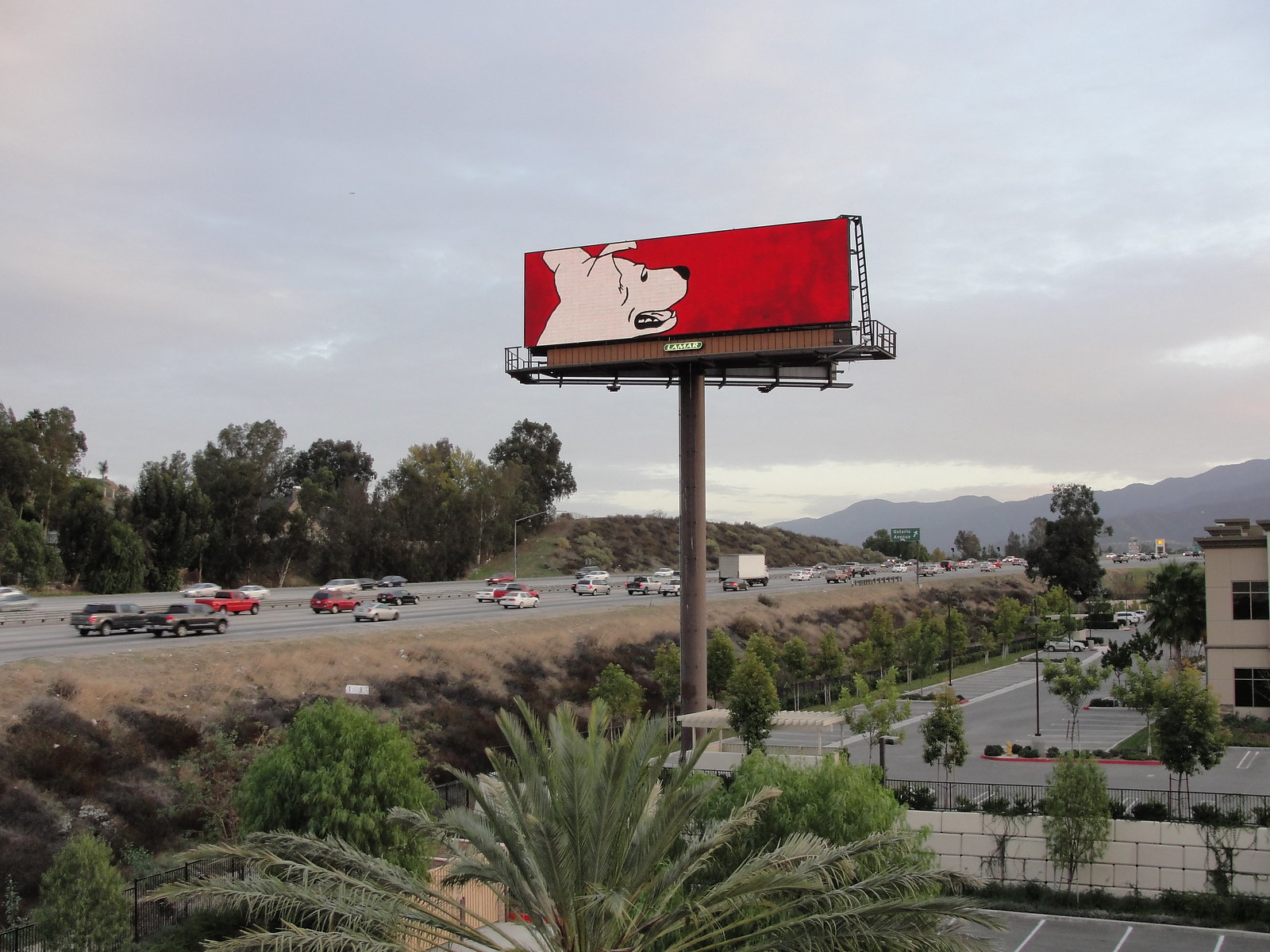The image showcases a large billboard prominently positioned beside a bustling highway. The billboard itself is strikingly red, featuring a tan and white dog gazing distantly towards the side. Numerous cars stream in one direction on the highway below, indicative of steady traffic flow. The sky above is overcast, casting a subdued and gloomy light over the scene. Surrounding the billboard and highway, there are abundant trees, creating a natural border. Distant mountains peek through the overcast, adding depth to the landscape. In the foreground, part of a building is visible; this structure is painted in a peach or off-white color, adding a contrasting architectural element to the natural surroundings.